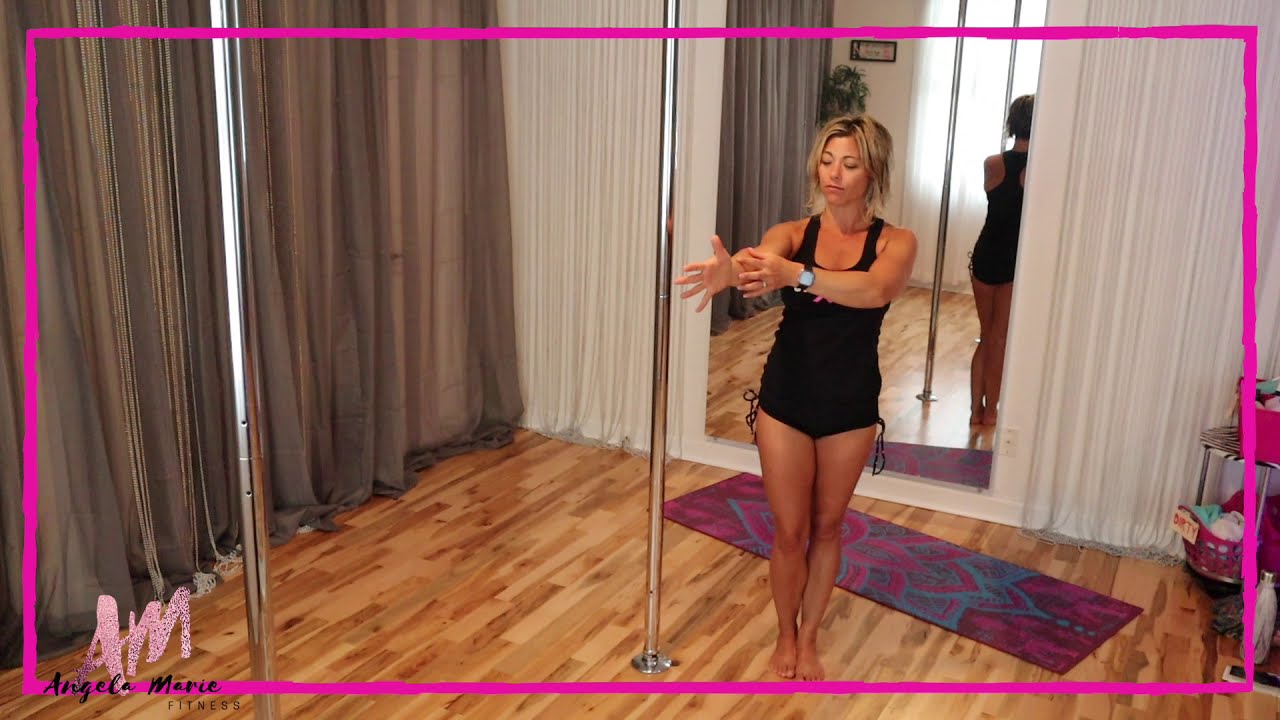This full-color, digitally enhanced photograph captures a woman in a dedicated indoor studio, possibly used for pole dancing. She is poised next to one of two silver-colored poles positioned in the center of the room, with her hands extended as if about to grab the pole. The woman has medium-length blonde hair, tied back, and she is wearing a black one-piece dress or a black tank top paired with very short black shorts. She is notably tan. The flooring is a rich, brown hardwood, and a yoga mat is laid out behind her. The walls feature a mix of dark brown and white curtains; the white curtain also houses a large mirror, reflecting the woman. The bottom left corner of the image features a logo consisting of the letters "A" and "M," with "Angela Mary Fitness" inscribed beneath. The entire photograph is framed with a pink rectangular border.